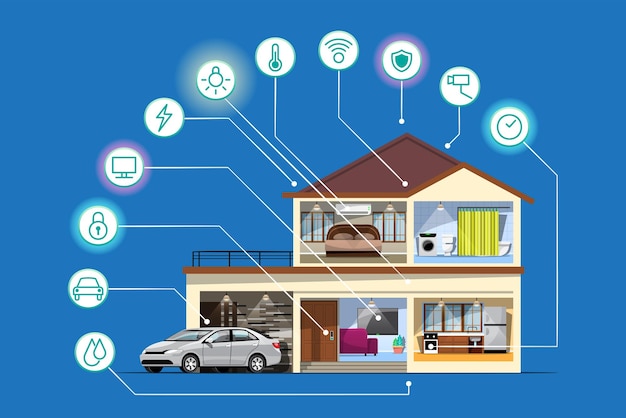The image is a detailed illustration of a two-story, cream-colored house with visible interior rooms, resembling a cut-out schematic design. The house has a dark brown A-frame roof and is set against a solid blue background. The ground floor features three square sections: a garage with a gray four-door sedan exiting diagonally to the left, a central living room, and a kitchen on the right. The upper floor includes two rooms: a bedroom with a bed and a bathroom with a yellow shower curtain. A triangular roof tops the structure, along with a beige border separating the two levels.

A series of white circles encircle the house in a flowing arc from the lower left to the upper middle and then down towards the right. Each circle contains an icon representing various smart home devices and utilities: a water droplet near the garage, a car near the sedan, a padlock near the entryway, a television, and a lightning bolt pointing to the roof, among others. Additional icons depict light bulbs, thermostats, Wi-Fi, home security cameras, and timers, some glowing blue or purple, indicating the range of technologies available in the house. The detailed captions and schematic layout showcase the smart home features integrated into each room of the house.